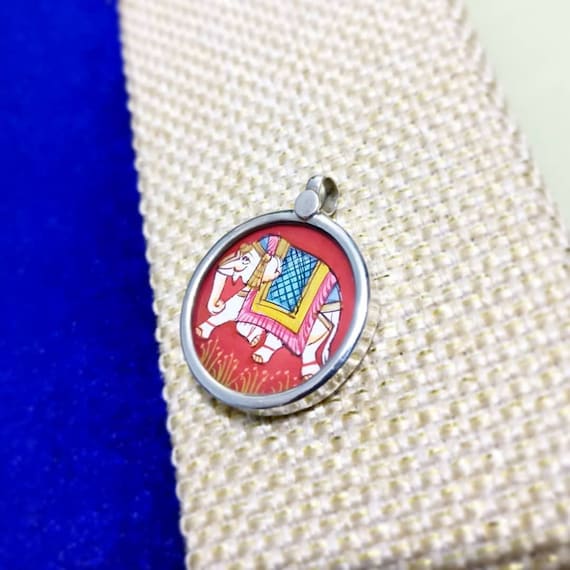The image features a detailed, round silver pendant resting on a folded, cross-hatched white mesh fabric. This fabric is positioned against a blue background on the left and a white wall to the right. The pendant itself has a high, shiny silver border and a small loop at the top. At the center of the pendant is a vibrant red background. Dominating the center is a simple yet elegant white elephant, which occupies about 70% of the pendant's face. The elephant is adorned with a decorative blanket on its back that features a pink trim at the edge, a yellow middle section, and a light blue center with a black diamond pattern. The elephant also has a scarf-like decoration around its head in matching colors of blue, pink, and yellow, with golden tassels hanging down. The bottom of the pendant's face includes painted dead brush and little green stems with tiny white buds, adding a natural element to the composition.